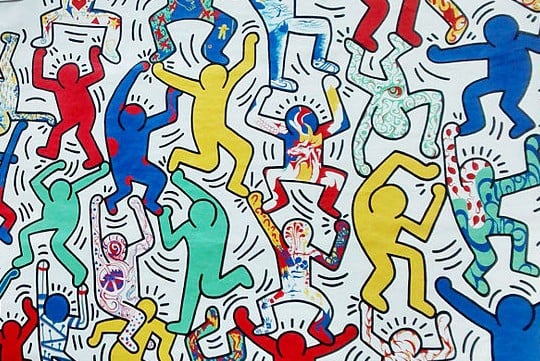This image depicts a vibrant, mural-like illustration of interwoven stick-figure-like cartoon people, dancing energetically against a solid white background. The figures, outlined in various bright colors such as blue, red, yellow, turquoise, and green, appear to be interconnected, celebrating a sense of unity and exuberance. Some of the figures feature unique patterns, including spots, squiggly lines, and zigzags, adding to the lively and dynamic composition. Their arms are outstretched, interlocking with one another, and they vary in size, creating a rhythmic and tiled visual effect across the artwork. The scene captures an essence of movement and communal connection.